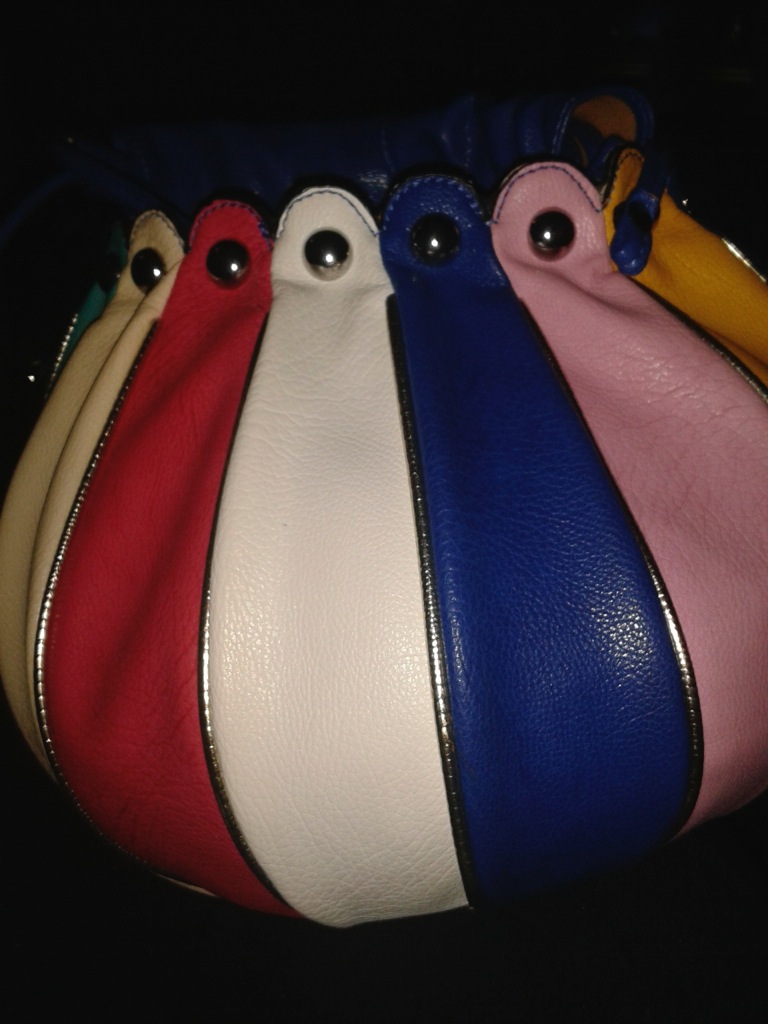The image depicts a spherical, multicolored bag, possibly a purse or satchel, adorned with vertical strips of faux leather in an array of colors. Starting from the left, the strips are green, beige, red, white, blue, light pink, and yellow, creating a vibrant mosaic. Each strip is bordered by black lines and joined together by a plastic-like material. At the top of each strip, there are round, silvery buttons, which may serve as a decorative element or potentially part of the closure mechanism. Additionally, the image shows the purse strap extending from the top, completing the distinct and detailed design of this unique accessory.